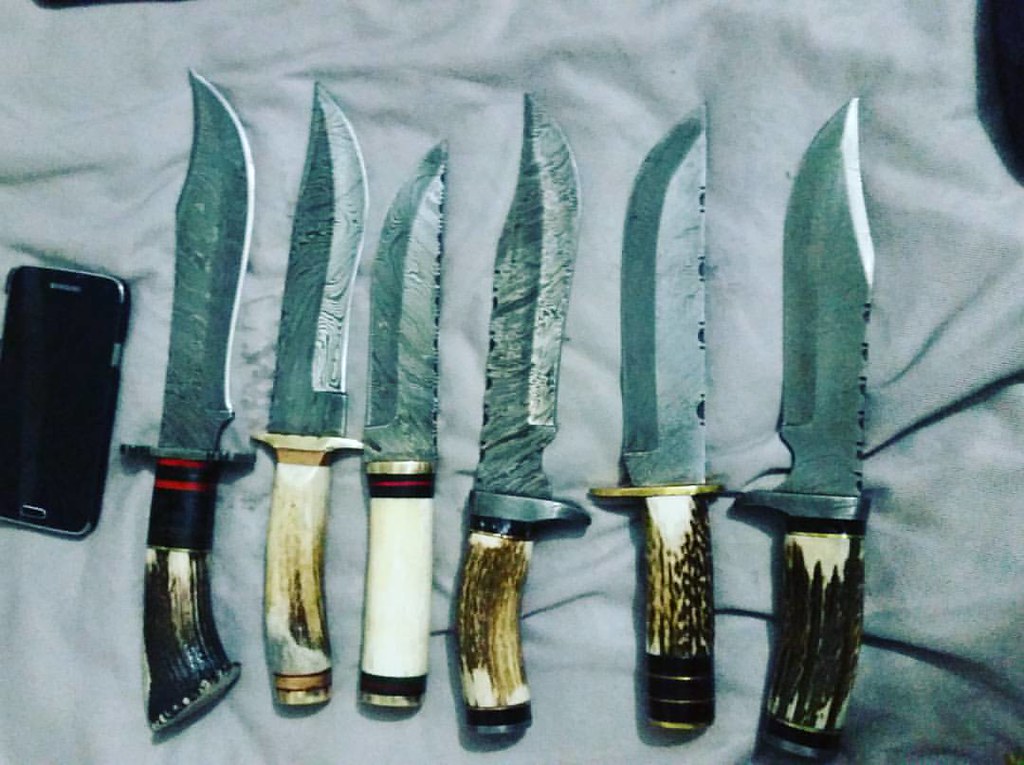In the image set against a light gray fabric, there's a smartphone placed on the left side of a bed. The phone, likely black, has its screen off, a brand or speaker slot on the top, and a button at the bottom. Spread across the bed are six large knives, each with distinct handles and sharp, pointed blades made of either silver, steel, or bluish metal. 

From left to right, the knives can be described as follows: 

1. The first knife has a black handle with ivory at the bottom and red straps in the center. The blade is long, curves downwards, and tapers to a very sharp tip.
2. The second knife features a white handle with brownish trim and a slightly curved tip.
3. The third knife sports a solid white handle with some brown stripes.
4. The fourth knife, marked by its brown handle accented with white, has a notably sharp and possibly curved tip.
5. The fifth knife has a predominantly brown handle with some white streaks.
6. The final knife has the darkest brown handle with a bit of white and a similarly large, sharp blade.

Each knife appears to be intended for use as a weapon rather than for kitchen tasks, suggesting a purpose such as hunting.